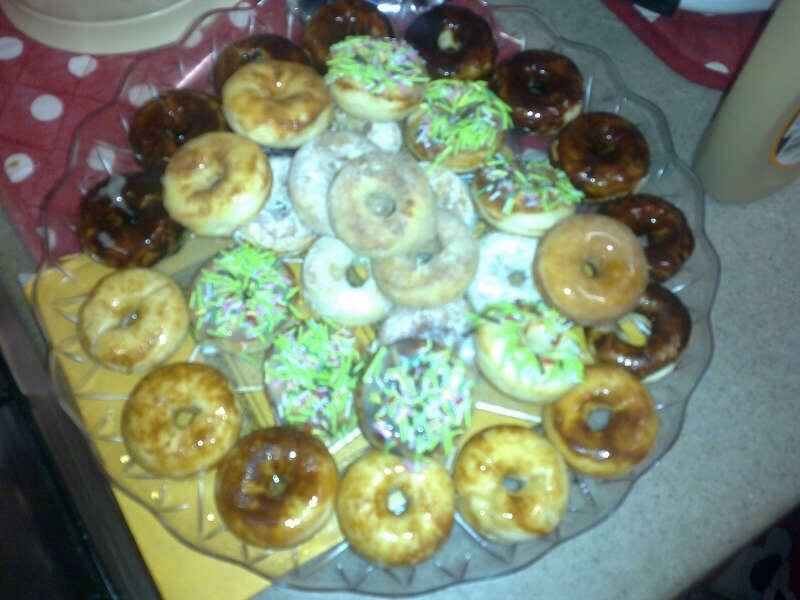In this overexposed photograph, a round glass platter is piled high with homemade donuts, arranged in a visually chaotic fashion. The platter sits on a speckled tan and white counter that is covered with a white tablecloth, accented by a yellow napkin and two red cloths with white dots. To the right of the platter lies a light tan bottle with an orange, black, and white label. The assortment of donuts on the tray includes various types: some donuts are coated in white powder, others are glazed, and a few are covered in chocolate frosting and adorned with a haphazard sprinkling of predominantly green sprinkles, interspersed with light red, white, and possibly blue bits. There are also donuts with a caramel-like drizzle and some with lime-green sprinkles. The flash used in the photo casts stark shadows, giving the donuts an unappetizing appearance that is further emphasized by the overall poor lighting, making the scene look rather unflattering despite the festive variety of the donuts.